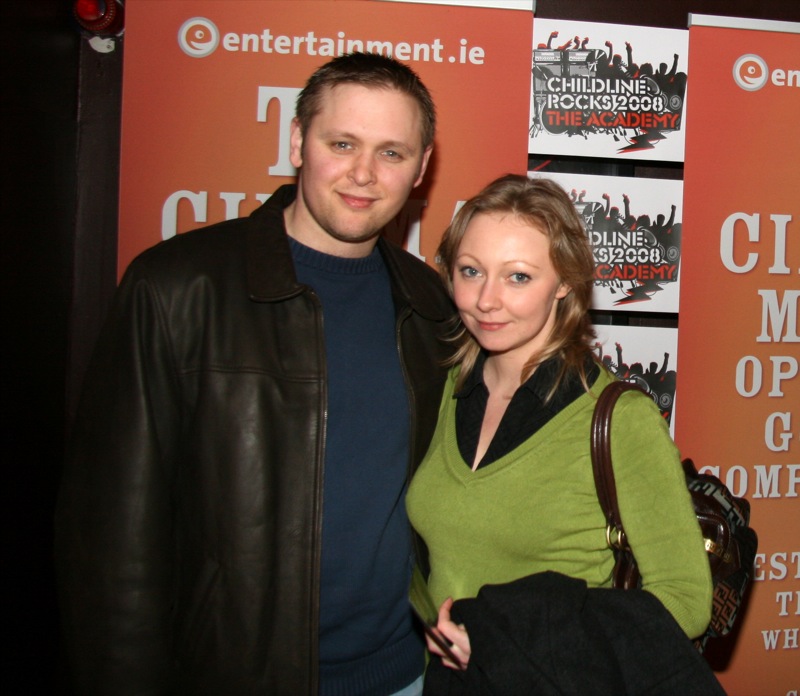The image features a man and a woman posing together in front of an advertisement board. The man, taller and positioned on the left, is a white male with dark blonde hair and blue eyes. He is dressed in a brown leather jacket over a blue t-shirt and blue jeans, smiling at the camera. The woman, shorter and standing on the right, is a white female with short, light brown to blonde hair and blue eyes. She is wearing a green v-neck shirt over a black button-down top, carrying a black coat or sweater over her left arm and a black backpack on her shoulder. They stand against an orange backdrop adorned with several logos and text. The prominent text reads "entertainment.ie" at the top, and includes "CHILDLINE ROCKS 2008" with "The Academy" in red underneath. The background also features an image of an excited crowd, creating an energetic atmosphere.